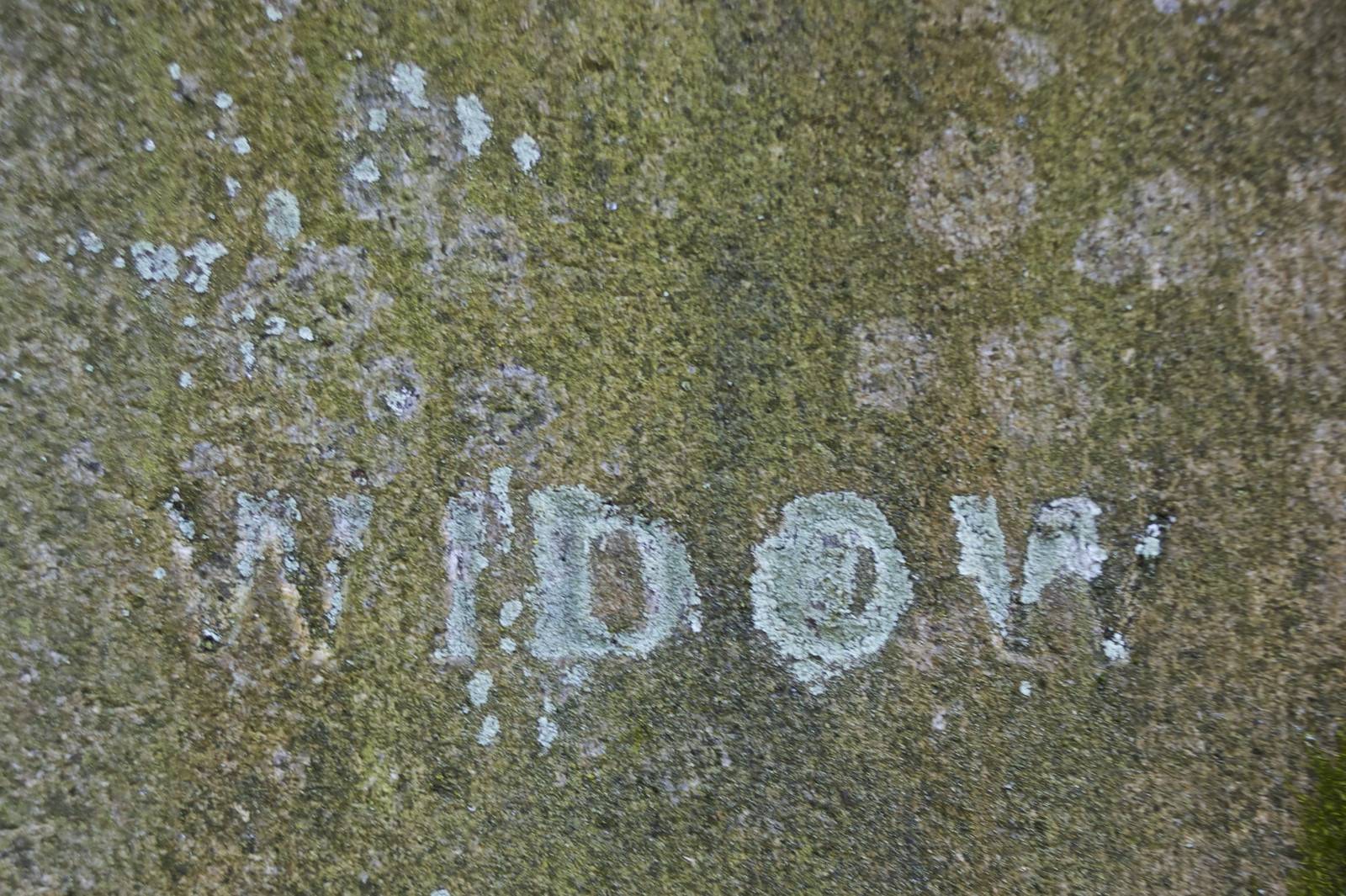This image, possibly a photograph, features a rectangular close-up view of what is likely a weathered tombstone or gravestone, heavily encrusted with algae, moss, mildew, and other ancient growths. The stone exhibits an off-green tinge interspersed with shades of yellow, white, gray, and black. The texture suggests a surface that one might pressure wash to remove the accumulated growths. Dominating the center of this image is the faintly etched word "WIDOW," partially filled in with the same algae and moss, which makes the engraving more discernible. The overall setting appears to be outdoors, likely in a cemetery, under daylight conditions. The details of the stone and its inscriptions are somewhat obscured by the layers of organic material, yet they hint at its memorial purpose.